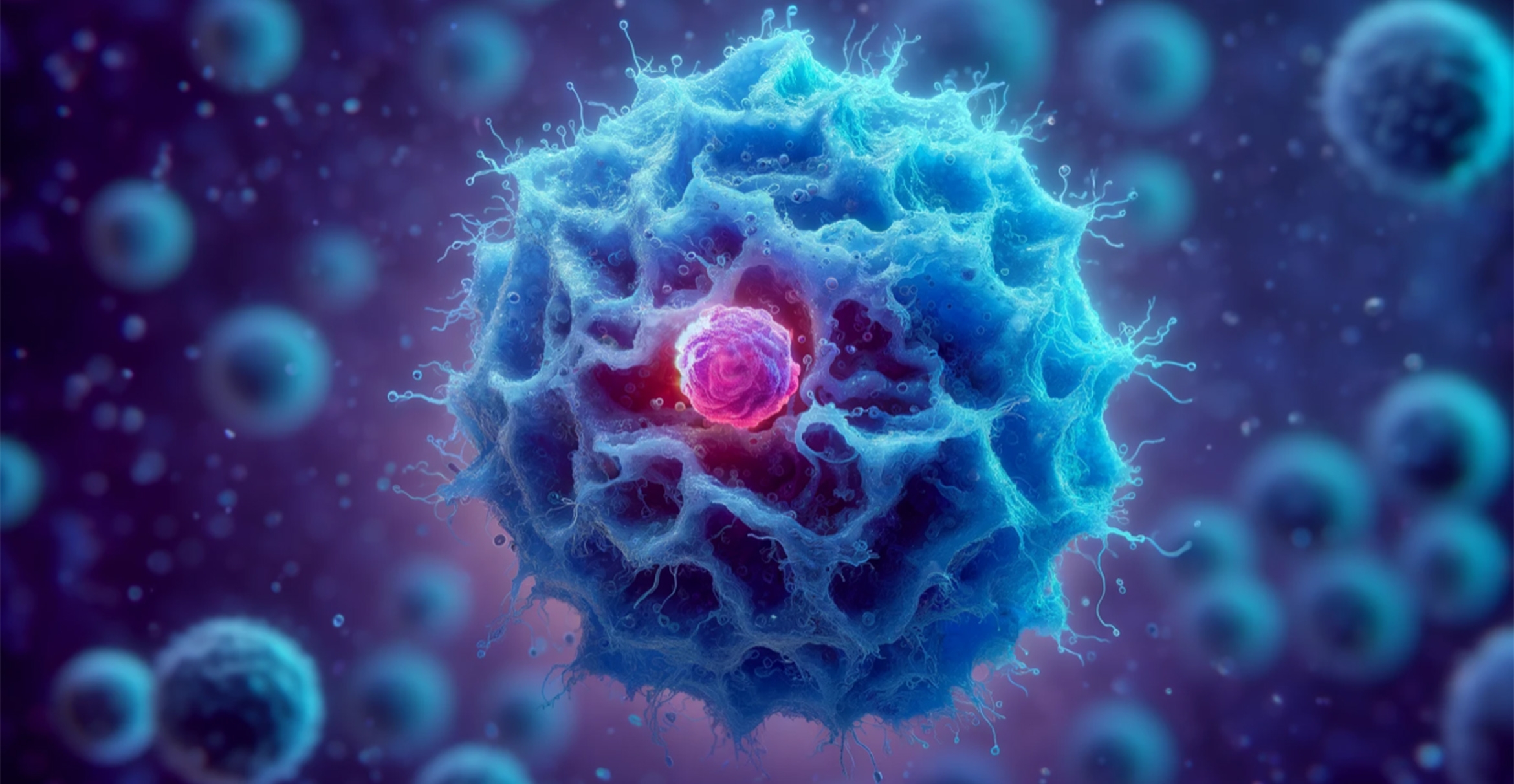This captivating digital art piece features a detailed, close-up view of a virus-like organism that bears a striking resemblance to the coronavirus. Dominating the center of the landscape-oriented image is a large, blue, circular virus structure. This main organism is adorned with intricate, thread-like extensions, some of which resemble sperm-like lines with small circles at their ends. Nestled within the heart of this blue virus is a smaller, vividly colored nucleus that transitions from red to pink, displaying a visually mesmerizing gradient.

Surrounding this central figure are clusters of similar blue, circular virus-like entities, scattered throughout the subtly blurred background to create a sense of depth and distance. The backdrop itself is a rich, radial gradient, transitioning from deep blue and purple on the periphery to lighter shades of purple and pink towards the center. This superbly crafted blend of colors enhances the focal pink nucleus, which also emits a faint hue, harmonizing with the overall color palette of the image. Scattered within this canvas are numerous tiny floating dots, adding to the microscopic feel of the scene.